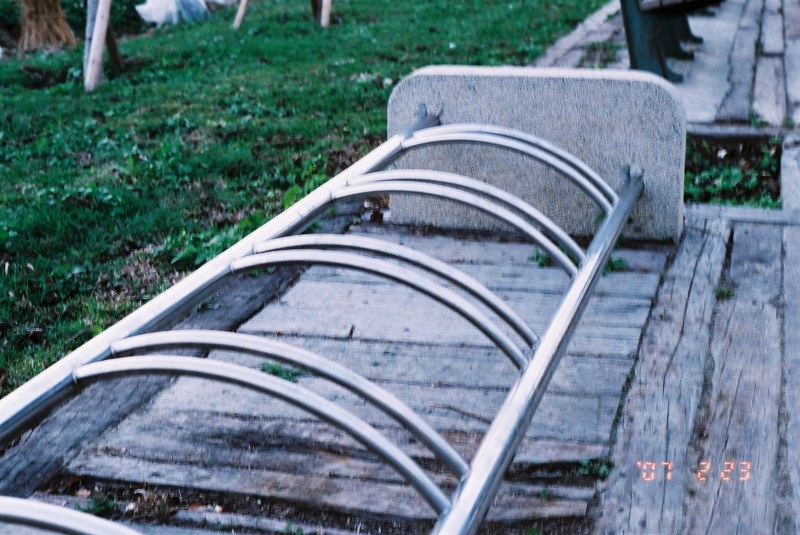This photograph, taken outdoors, showcases an empty silver chrome bike rack with two long parallel pipes connected by curved metal bars, standing on a weathered wooden platform. The wood planks, greyed and rotting, form the ground base beneath the bike rack. Surrounding the rack is a patch of plush, darker green grass, extending to the left side of the image. Partially visible in the scene is the trunk of a tree, planted within a concrete holder adjacent to the wooden base. In the bottom right corner of the image, there are orange digital numbers "07223," reminiscent of a clock display. The perspective of the photo is from above, providing a clear view of the entire setup.